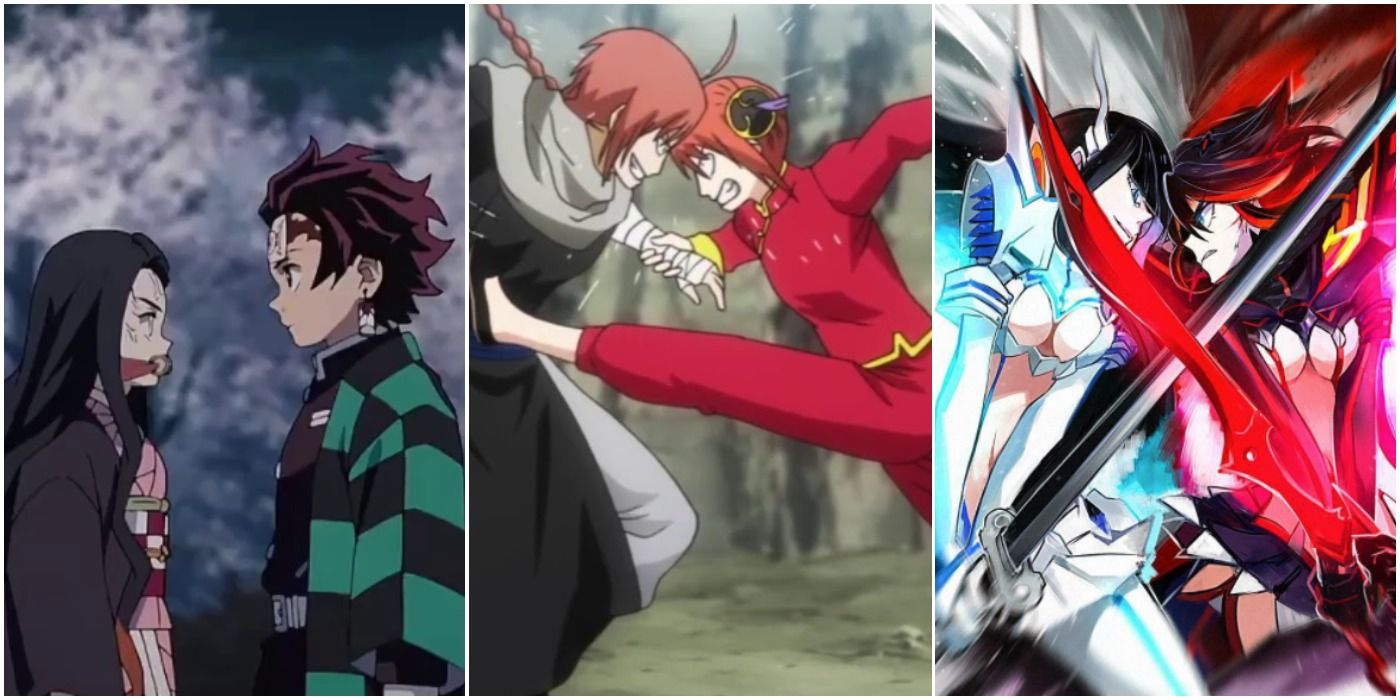The image is a detailed triptych featuring three distinct scenes from popular animes of the 2010s to 2020s, each showcasing pairs of sibling characters. On the left is a dynamic screenshot from "Demon Slayer," depicting a boy with burgundy-black hair and green and black attire, staring intently at a girl with long black hair. She has a furious expression, and the nighttime setting is accentuated with a blurry backdrop that appears to be cherry blossom trees. Notably, the girl has something tied around her mouth, preventing her from speaking.

In the center, a fierce battle scene from "Jintama" is captured, showcasing two women with striking red hair. The woman on the left, cloaked in black, faces off against her sibling, who is clad in a vivid red outfit. The red-clad character is mid-kick, aiming at her opponent, portraying an intense moment of conflict.

The rightmost image, which might be a promotional image from "Kill la Kill," vividly illustrates two scantily clad sisters in an intense swordfight. Both women, though minimally dressed, are fully armed and locked in a face-to-face standoff, their expressions and postures brimming with animosity. The sister on the left dons blue and white, while her counterpart is dressed in vibrant red. Each scene, though differing in art style, captures the dramatic essence of sibling rivalry pervasive in these animes.